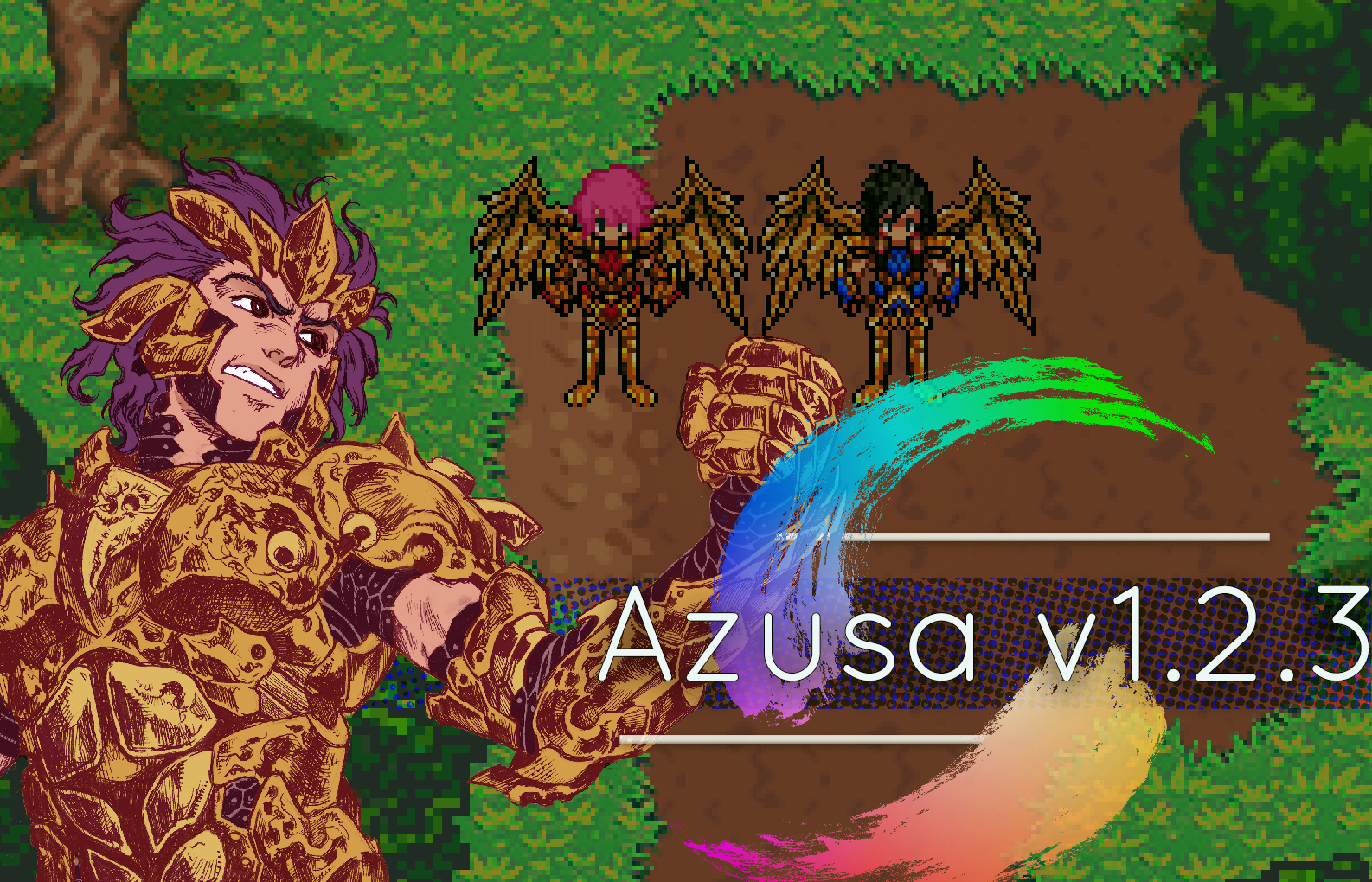The image appears to be a computer-generated scene, likely from a video game. The background is an 8-bit or 16-bit style with a green field and a dirt area. Across the dirt, white text reads "Azusa version 1.2.3," framed above and below by swirls of color. On the left side of the image, dominating the scene, is an anime-style warrior with purple hair and a grimace, clad in heavy, gold-plated armor with brown accents. His fist is raised in the air, emphasizing his fierce demeanor. Behind him, two gargoyle-like creatures with brown wings and armor stand on the dirt. The creature on the left has pink hair, while the one on the right has dark green hair. These creatures, though similarly armored, contrast sharply with the central warrior figure and appear integrated into the green and brown 8-bit landscape.